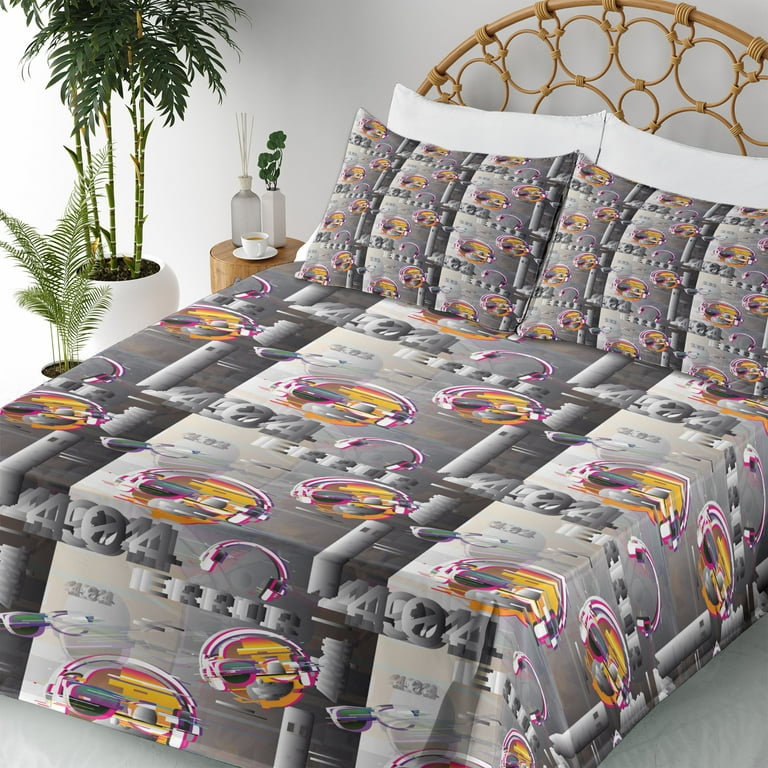The photograph showcases a serene bedroom characterized by its white floors and walls. Dominating the image is an inviting bed adorned with a large circular rattan headboard, featuring small, intricate circles within its bamboo-colored framework. The bedding ensemble includes a gray comforter and pillow set, detailed with two shades of gray and accented with a colorful, futuristic ball displaying shades of yellow. Leaning against two pristine white pillows are additional pillows featuring a unique pattern of reddish magenta and white headphones, complemented by a whimsical design that seemingly includes a yellow head and green lenses within the pattern. Beside the bed sits a wooden nightstand holding a reed diffuser, a white vase with green flowers, and a teacup filled with light brown liquid. Completing the tranquil setup are two potted plants, one with a white vase hosting tall greenery, creating a calm and inviting sanctuary.